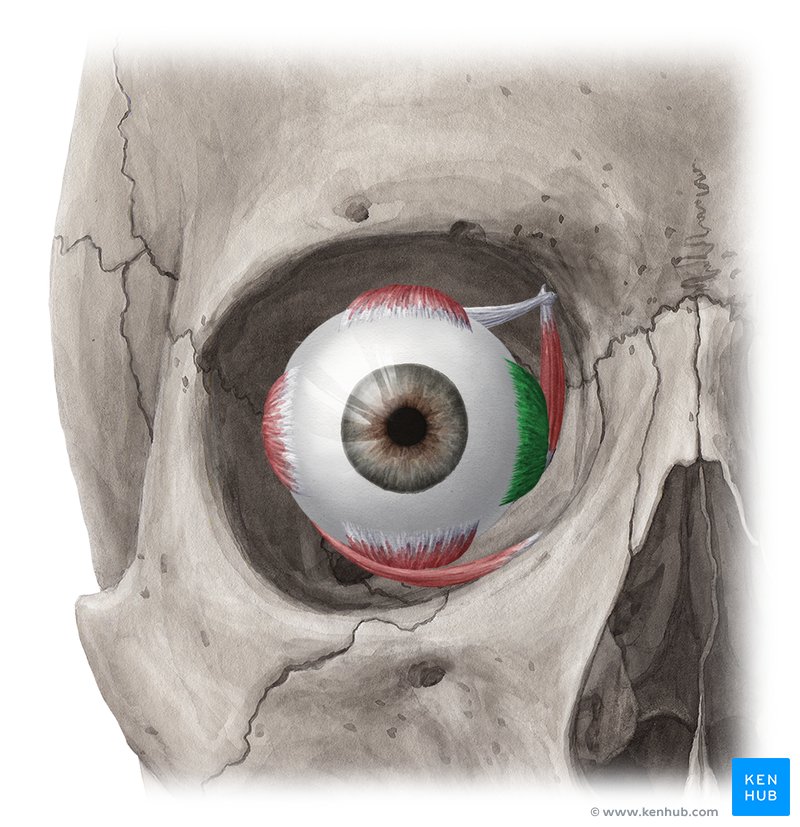This detailed painting or illustration presents a close-up of the right side of a human skull, facing the viewer, with a semi-realistic eyeball intricately drawn into the eye socket. The skull itself is depicted in shades of gray and white, featuring detailed cracks and highlighting the structure of the nose cavity. The focus is primarily on the eye socket, where the eyeball appears with a brownish-gray iris, surrounded by specks of red on the top, left, and bottom, and green hues on the right side. The illustration meticulously portrays the eye's connective tissues and nerves extending into the skull. On the bottom right of the image, there is a small blue box containing the text "Kenhub" along with the website "www.kenhub.com".